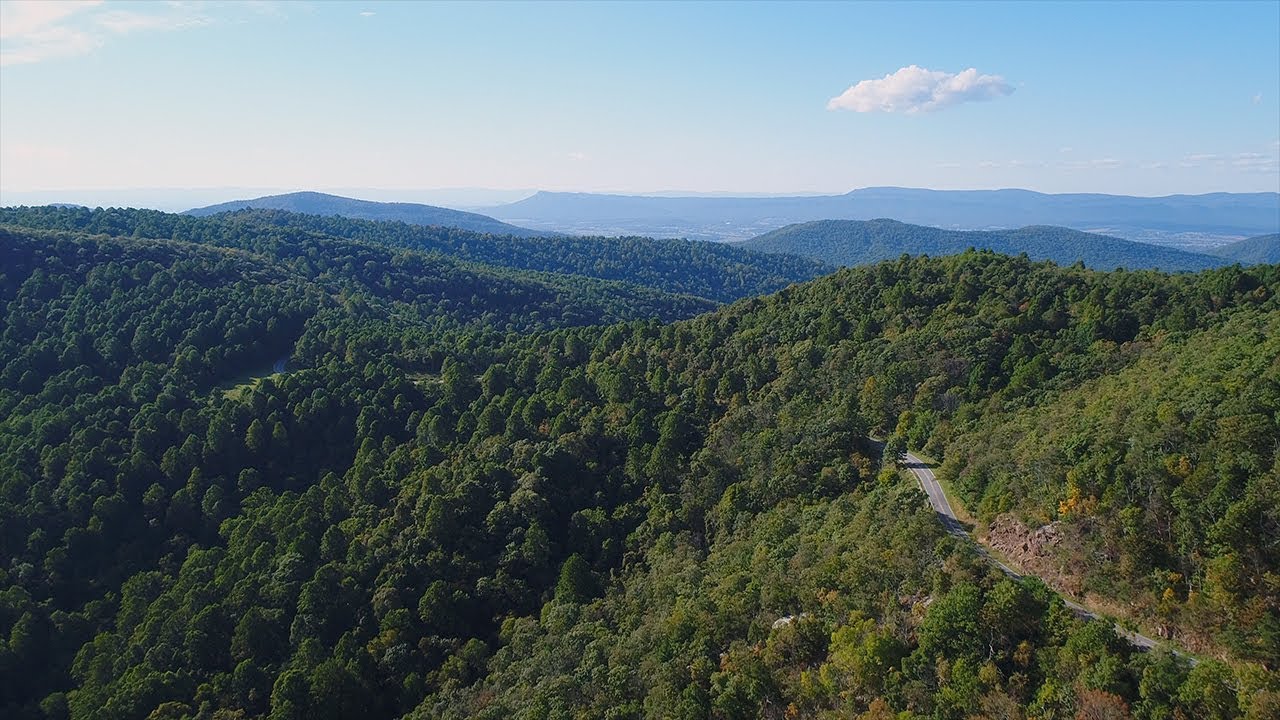The landscape photograph captures an expansive, undetermined location dominated by rolling hills densely covered with green trees, ranging from stunted scrub oaks to taller varieties, extending endlessly into the horizon. The scene is bathed in natural sunlight, creating a hazy, distant effect. A lone, white, fluffy cloud floats in the top right of the clear blue sky, with another cloud visible in the upper left. The bottom right of the image features a solitary two-lane paved road, marked by a yellow dividing line, which starts from the bottom left corner, winds through the hills, and frequently disappears into the dense foliage before reappearing further along its route. Far in the distance, one might faintly discern the silhouette of a city, although the overwhelming focus is the vast, undisturbed sea of green trees punctuated only by the meandering road and the vast sky above.